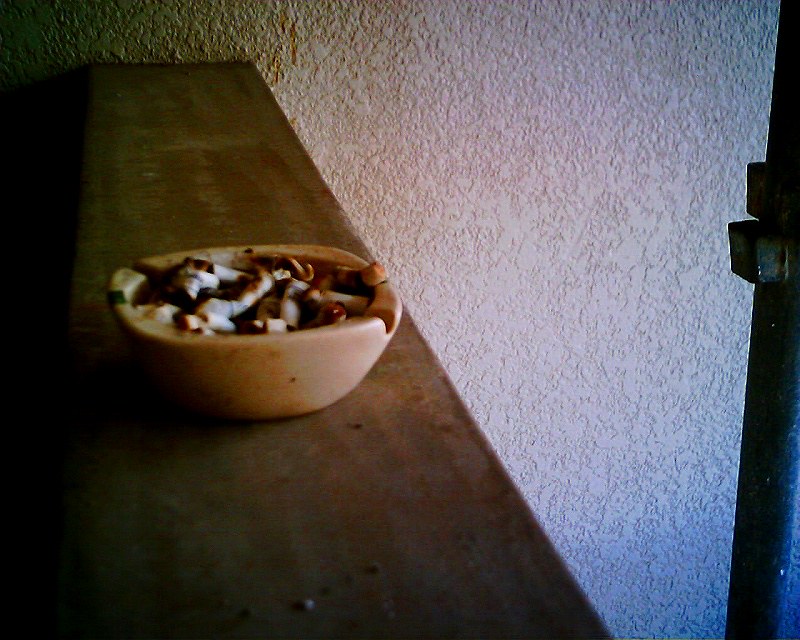The photograph depicts a tan ceramic bowl, functioning as an ashtray filled with numerous cigarette butts, resting on a flat-topped wooden railing. The bowl features grooves along its side, presumably for resting cigarettes. The setting appears indoors, illuminated dimly, with shadows cast across the table and the bowl. The railing, which is brown, is positioned against a white, textured plaster wall that resembles either a popcorn or eggshell finish. The bowl is placed just left of center on the railing. The color palette consists mostly of neutral tones such as brown and tan, with no additional text or objects present in the background to detract from the scene’s simplicity.